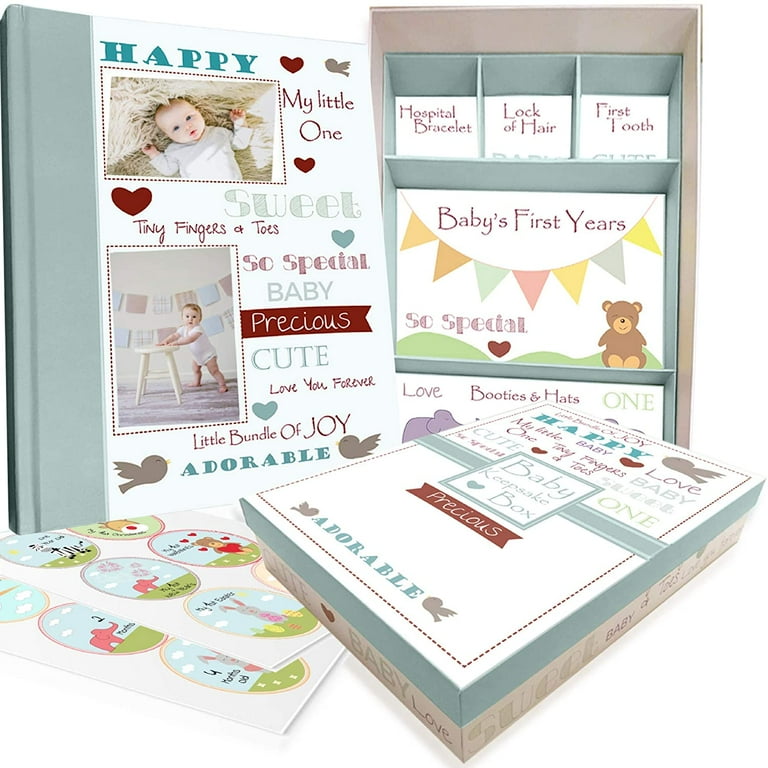The image captures a delightful baby book and keepsake kit against a white background. On the left is a baby book with a sage green binding and a white cover, featuring two charming photos of infants: one lying on a fur rug looking up at the camera, and the other standing while holding a small white stool. The cover is adorned with text in various fonts and colors, reading "Happy," "My Little One," "Sweet, Tiny Fingers and Toes," "So Special," "Baby," "Precious," "Cute," "Love You Forever," "Little Bundle of Joy," and "Adorable," alongside hearts and tiny cartoon bird silhouettes.

To the right of the book lies the interior of a keepsake box with compartments labeled for special mementos like "Hospital Bracelet," "Lock of Hair," "First Tooth," and a central section titled "Baby's First Years," decorated with a teddy bear and bunting. Below, the matching cover of the keepsake box echoes the book's design and phrases such as "Happy," "My Little Baby," "Love," "Baby Keepsake Box," and "Adorable."

In the bottom left corner, two sheets of circular milestone stickers featuring cute cartoon elephants and rabbits are visible, intended for marking the baby's growth and achievements. Together, the book and keepsake box offer a charming way to preserve precious memories of a baby’s early years.